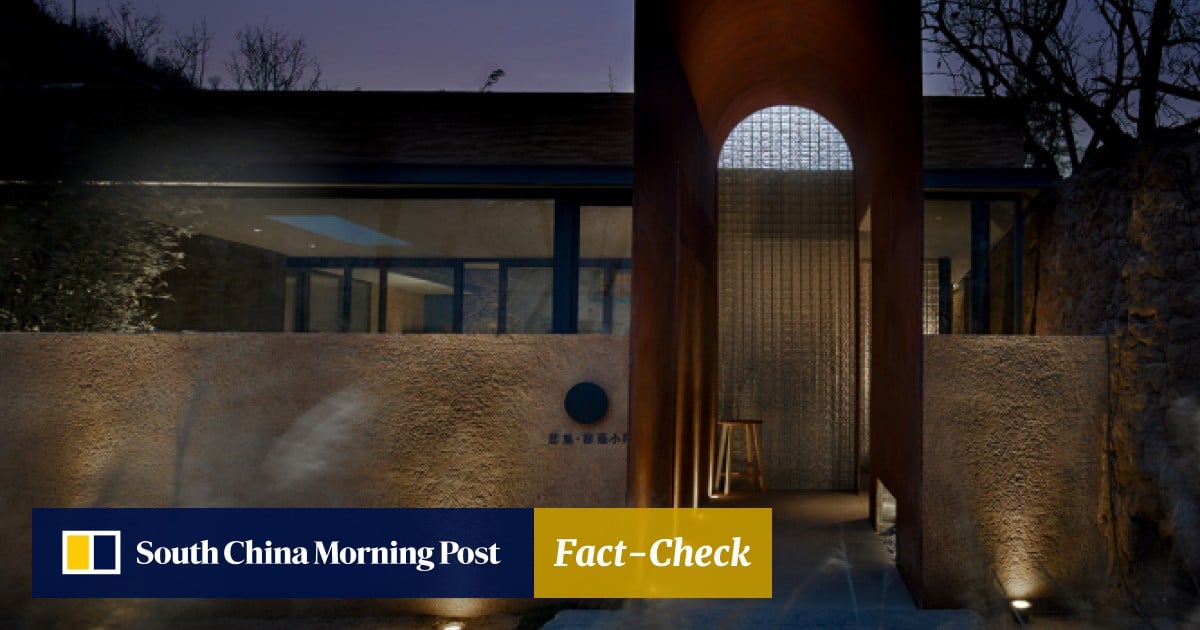The image depicts an elegant and modern architectural design of a building entrance, captured during the evening. The main entrance features a tall, curved, and smooth brown structure, which is illuminated from below to accentuate its shapes. A glass door with a vertical line pattern is visible behind this structure. The surrounding walls have a textured appearance, likely made of stone or a similar material, with subtle lighting that enhances the aesthetic appeal by illuminating part of the wall and ground. The background shows dim lighting with a dark sky, indicating it is nighttime. Trees and tree branches frame the building on both sides, adding a touch of natural elements to the modern design. Positioned at the bottom of the image is a piece of text reading, "South China Morning Post Fact Check," with a background of yellow and dark navy blue. The building, which appears to be either a place of business or a home, is beige with a black roof. The overall setting is decently lit, providing a clear view of the modern architectural elements and surrounding environment.